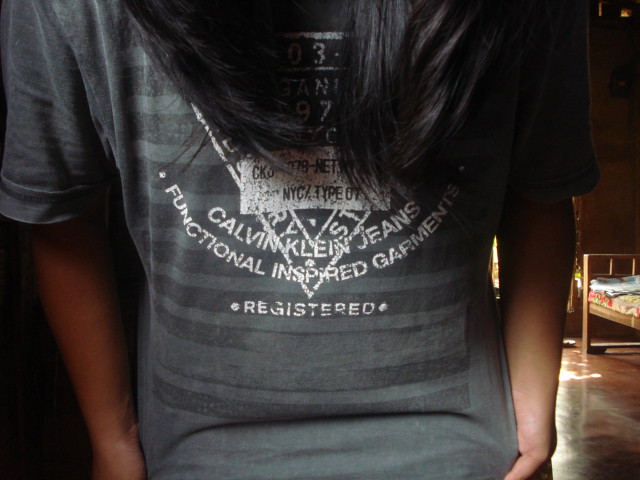This color indoor photograph, taken during daylight, features a single individual with long straight black hair, partially obscuring their face and upper body. The person is slightly bending forward, showcasing their gray Calvin Klein t-shirt emblazoned with the phrase "Calvin Klein Jeans Functional Inspired Garments Registered," though some of the text is partially obscured by their hair and hand placement. The background reveals a wood floor illuminated by light streaming through a window, and a modest single bed adorned with a floral print and either a very flat pillow or folded sheets at its foot. Black and gray striping elements are also visible in the surroundings. The composition resembles an upside-down triangle due to the person's pose and the way they hold the shirt downward to display it.